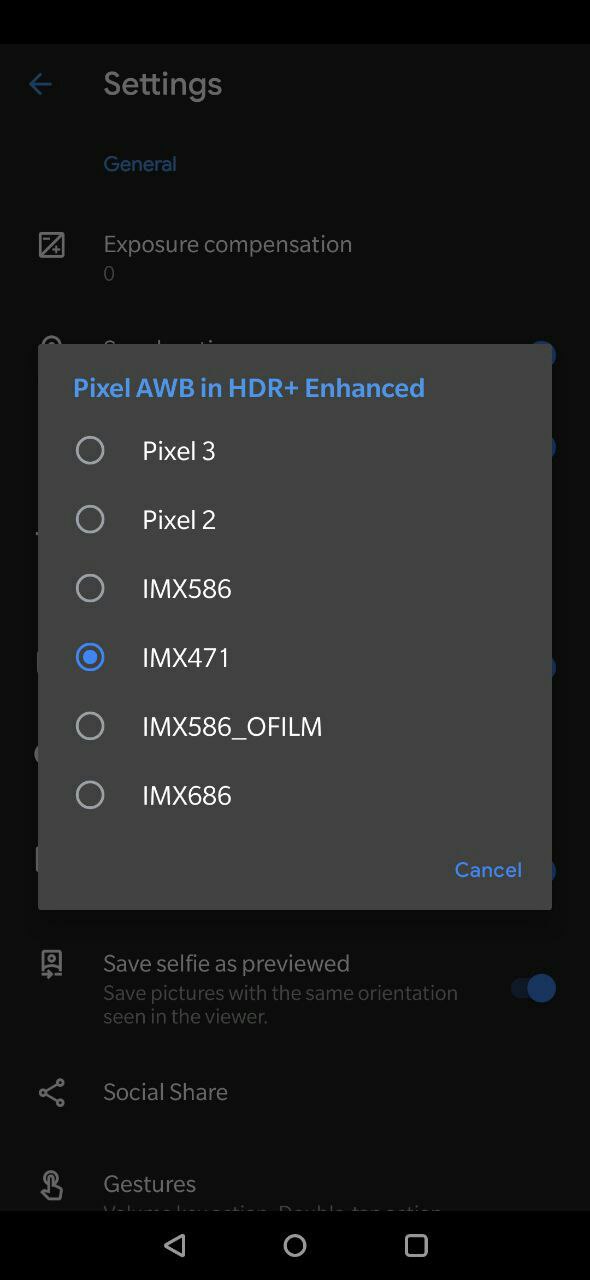The image depicts a mobile phone interface focused on a "Settings" menu. The screen's height is elongated, fitting the full width of the display. The top portion of the screen is partially obscured, although "Settings" is identifiable at the top. To the left of "Settings," there is a left-pointing arrow, appearing blue but slightly faded due to an overlay. 

Below "Settings," the word "General" is visible and highlighted in blue. Directly underneath "General," the term "Exposure Compensation" is displayed with an adjacent option box. This box contains a minus sign and a plus sign, divided by a diagonal line. Beneath "Exposure Compensation," a small zero is displayed next to another gray selection box.

In the middle section, the screen reads "Pixel AWB in HDR+ Enhanced" in bolded blue font. Below this, several empty circular selection options are shown, with only one option marked as selected: "IMX471." The other options remain unchecked.

At the bottom right corner of the overlay, the word "Cancel" is presented in blue font. The entire overlay appears as a slightly transparent gray box, giving a scraped appearance.